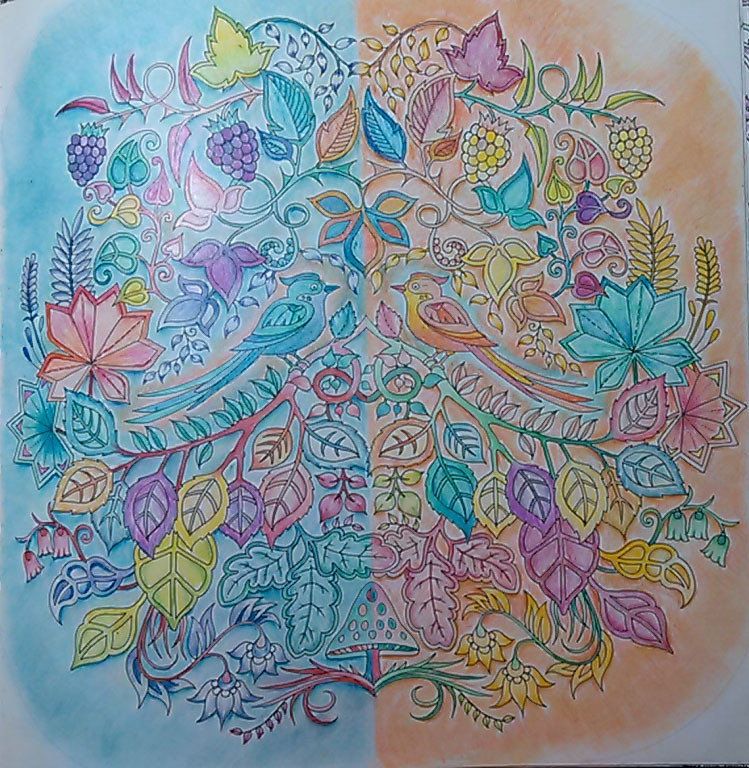This vibrant artwork showcases a captivating, dual-toned design, split between teal on the left and blue on the right. Each side features a bird perched on a branch, painted to match the dominant color of its background while being enveloped in hues from the opposite side. The branches, adorned in green and pink, are festooned with a stunning array of leaves and flowers in every color of the rainbow. Among these, small clusters of grapes stand out, with yellow grapes on the teal side and purple ones on the blue side. This detailed piece bursts with vivid, varied colors, creating a mesmerizing and beautiful visual experience.